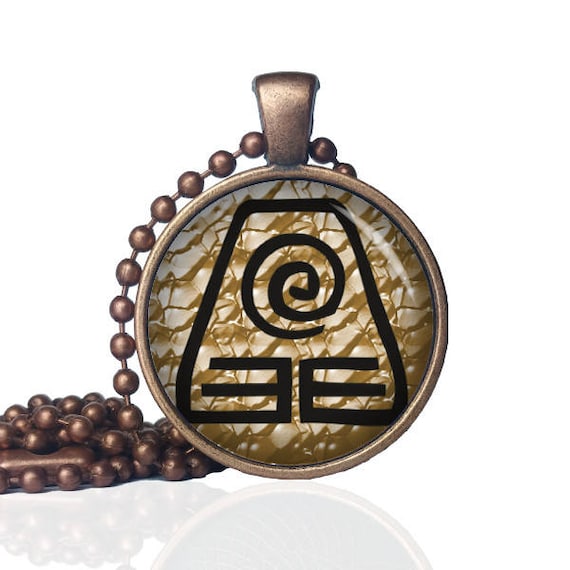The image showcases a pendant and chain with intricate details. The pendant is large, round, and framed by a dark brass-colored metal. The design within the pendant features a prominent black insignia from the Avatar movie, characterized by a distinct hieroglyphic symbol resembling an upside-down V, which extends into three horizontal lines with a swirl at the top center. The backdrop of the insignia is a white and gold swirl marble pattern that mimics cracked sand or glass. The pendant has an opening at its top for a chain, which consists of small, shiny round beads connected in a chain-like fashion. This chain is gathered and puddled on the left side, though no surface is visible. The detailed composition gives the pendant a vintage aesthetic, reminiscent of an old-fashioned watch, complemented by its brass metal tone and reflective shine.